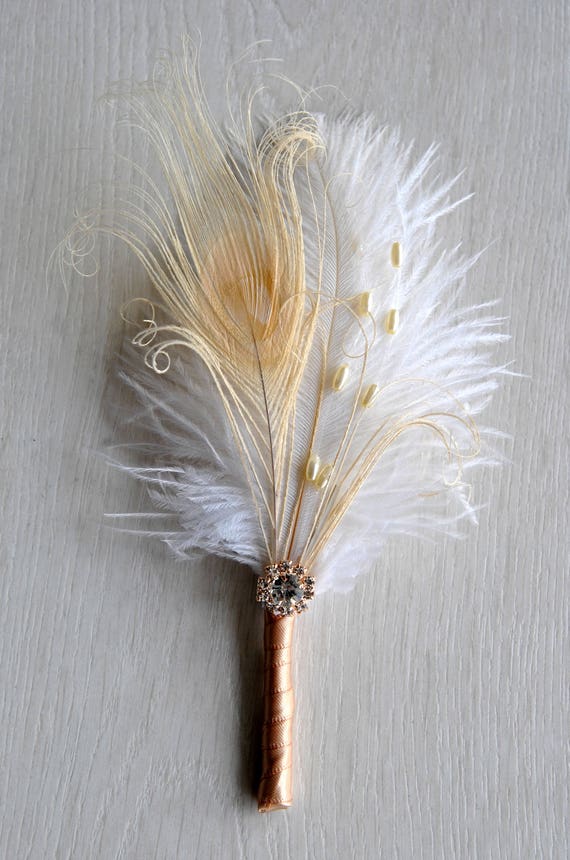The image depicts an ornate feather arrangement resting on a painted white wooden surface. The central focus is a collection of plumes intricately embellished and stylishly presented. The feathers, primarily white and gold, include a standout gold peacock feather positioned among fluffier white feathers at the back. In contrast, the front features sand-colored feathers with delicate curls at the ends. Enhancing the composition, pearl-like, pill-shaped beads are interspersed on the right side of the white feathers, adding a touch of elegance. The stems of the feathers are tightly bound in a shiny, creamy gold or rose gold ribbon, extending halfway up and creating a refined look. At the feather base, a brooch adorned with black or gray gemstones, set in rose gold metal, adds a lavish touch, amplifying the decorative appeal of the arrangement. The image's plain background, described variably as beige or white, provides a stark contrast that accentuates the intricate details and lustrous elements of the feather decoration.